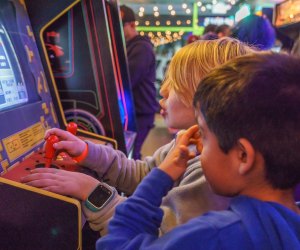The image captures a lively scene at an arcade, where two boys are immersed in a retro gaming experience. The blonde boy, dressed in a sweatshirt and an Apple watch, is fully engaged in playing a game with red joysticks on a black arcade cabinet highlighted with gold trim. Beside him, a brown-haired boy in a blue hoodie observes while scratching his eye. The arcade room is buzzing with activity; neon lights illuminate multiple gaming machines, including one with an orange joystick up close and another with a green joystick further back. Various people are dispersed throughout the room, indulging in their own games under the arcade's atmospheric gold and green lighting. The surrounding machines and their colorful outlines add to the nostalgic ambiance, possibly hinting at classic games like Tetris.